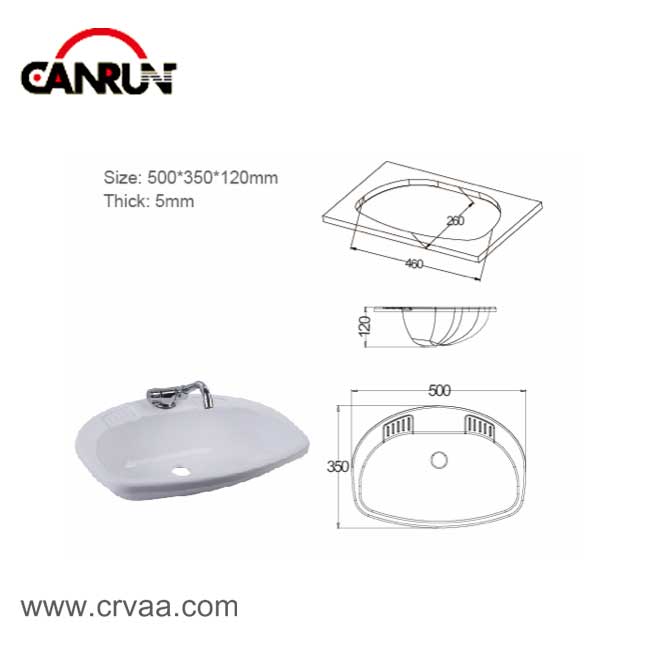The image features a detailed photograph and various line drawings of a white porcelain sink with a silver faucet. The top left corner displays the brand name "CAN RUN" in black letters, with a red arch above it. Below the brand name, black text reads "SIZE 500 x 350 x 120 mm" and "THICK 5 mm." Further down, in gray text, is the website "www.crvaa.com."

On the lower third of the image, the photograph of the sink prominently stands out. To the right of the sink, there are three black-and-white line drawings illustrating its dimensions and shape. The top drawing is a rectangular surface with a hole meant for the sink, measuring 460 mm wide and 260 mm tall. The middle drawing depicts a cross-sectional view of the sink, showing a half-sphere depth of 120 mm. The bottom drawing presents an overhead view, illustrating the complete sink with a horizontal width of 500 mm and a vertical height of 350 mm. This drawing includes details such as the circular drain in the center and two grooves for soap at the top. The entire image is set against a white background, providing a clear and clean presentation of the sink and its schematics.